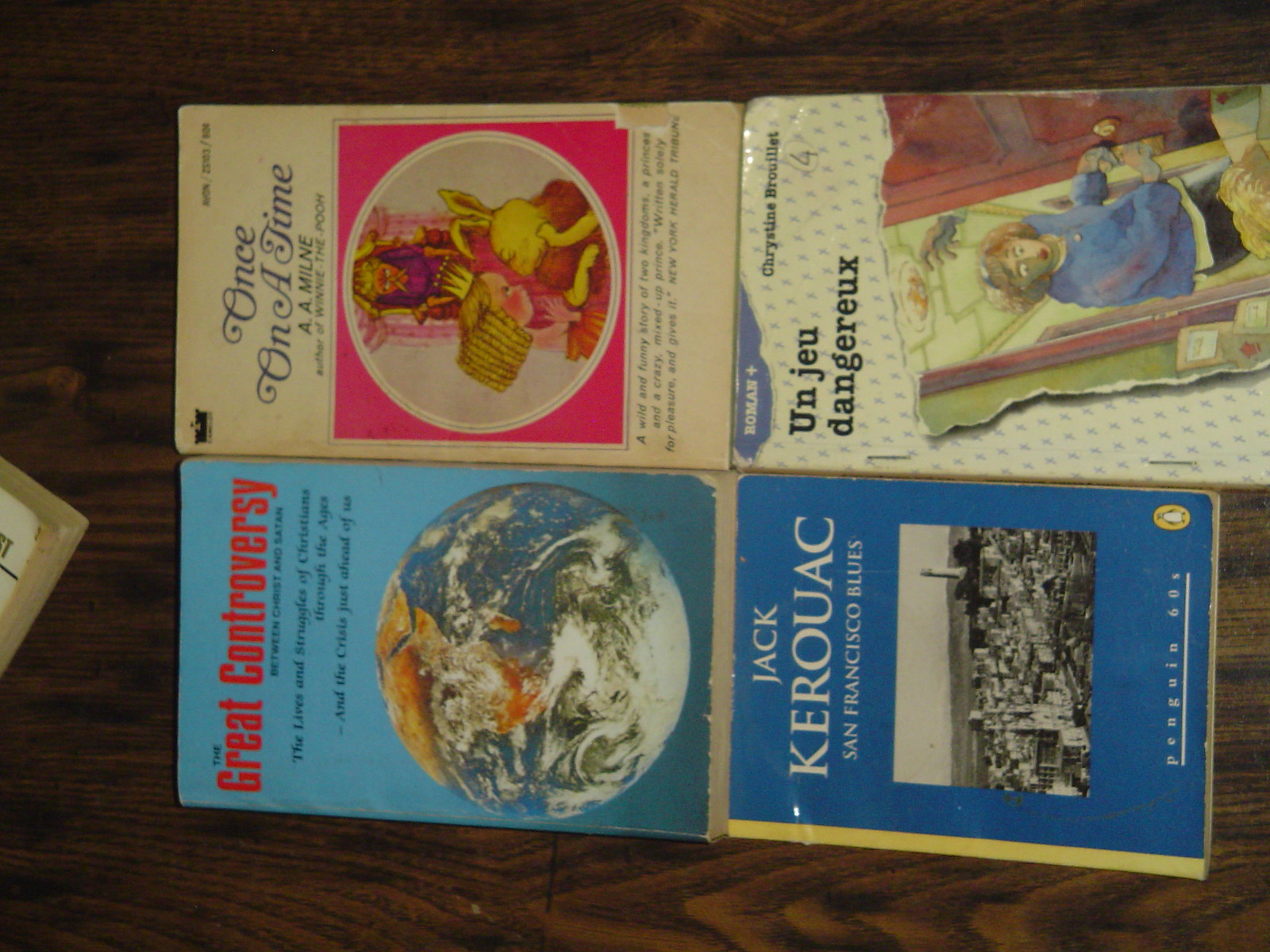This detailed photograph, taken from above, showcases four old paperback books placed on a dark, reddish-brown stained wooden table, arranged side-by-side in two rows of two. The first book on the upper left is titled "The Great Controversy," featuring a blue cover adorned with an image of the Earth, showcasing visible clouds and bodies of water. Adjacent to it, on the upper right, is "Once on a Time," a cream-colored book with a central pink square that encloses an illustration of a princess or queen conversing with a human-like rabbit. Below "The Great Controversy," in the lower left, is "The San Francisco Blues" by Jack Kerouac, which presents a cityscape on a dark cover. The final book, positioned to the right of Kerouac's, is a foreign language paperback featuring a white cover with light blue dots, depicting a woman looking downward while opening a door.